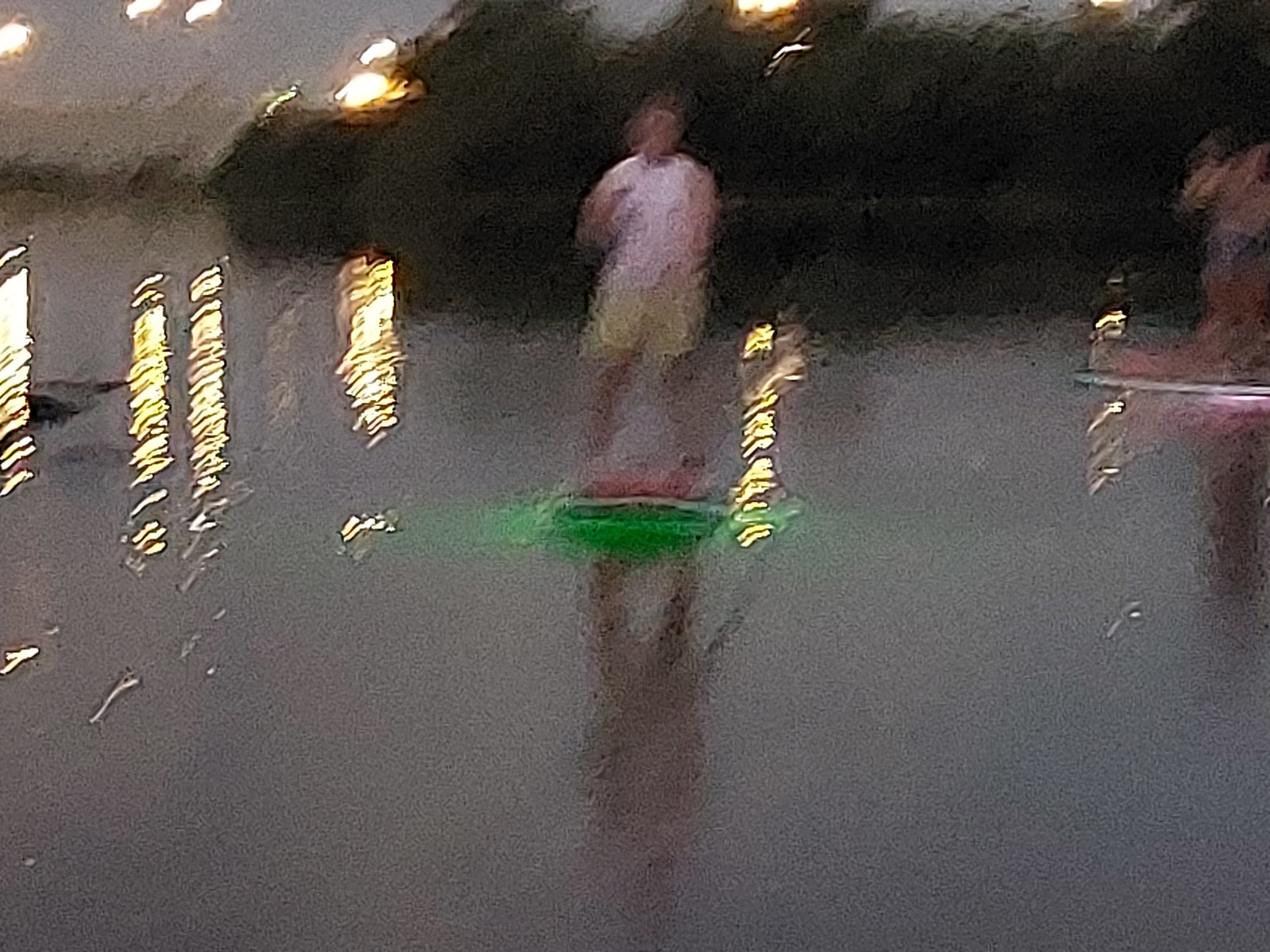The image is a blurry, overexposed photograph featuring a person standing on a surface that reflects light, suggesting it could be water or wet pavement. The person is wearing yellow shorts and a pink or white short-sleeved shirt, with tan legs and black hair. They appear to be standing on a board or platform that is illuminated with green light and has red edges. Scattered throughout the photo are horizontal lines and rectangular light reflections, adding to the overall confusion of the scene. There are also yellowish streaks and possible reflections of another board with a figure possibly in the upper right corner, contributing to the notion of an outdoor setting, perhaps on a rainy day with an art-like effect applied to the image.